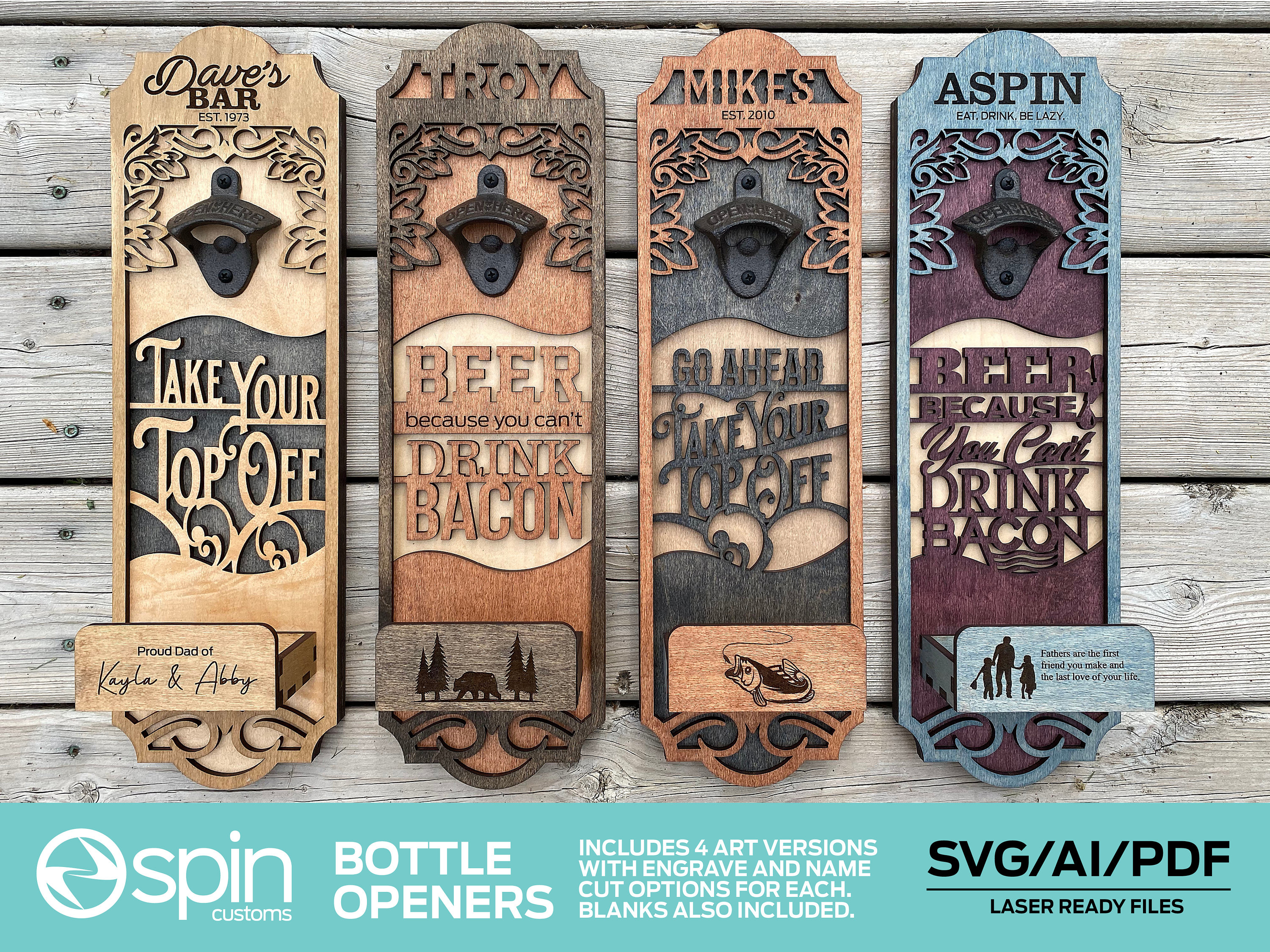This advertisement for Spin Customs showcases four personalized bottle openers, beautifully crafted with laser-cut wooden planks and metal opening mechanisms. The Spin Customs logo, a circle with intertwined swooshes resembling boomerangs, is prominently displayed in the lower left corner within a light blue footer that spans the bottom of the rectangular, outdoor photograph. The text in the footer details that the product includes four art versions with options for engraving and name cuts, as well as blank versions. Additionally, the files are available in SVG, AI, and PDF laser-ready formats, ensuring that each design can be tailored to individual preferences.

Against a backdrop of aged gray wood panels, the four distinct bottle openers are highlighted, each varying in color and design. The first opener features a light yellowish tone with the phrase "TAKE YOUR TOP OFF" in its center and reads "DAVE'S BAR, Established 1973" at the top. The bottom inscription celebrates family with "Proud Dad of Kayla and Abby." The second opener, with an orangish-brown hue, sports the humorous quote "BEER BECAUSE YOU CAN'T DRINK BACON," accompanied by a bear and tree illustration. The third, dark-toned opener says "GO AHEAD, TAKE YOUR TOP OFF" and includes an image of a fish leaping towards a worm. Above it is the personalization "MIKE'S, Established 2010." Lastly, the blue and mauve opener also displays the beer and bacon quote and features the text "ASPEN, EAT DRINK BE LAZY" at the top and "FATHERS ARE THE FIRST FRIENDS YOU MAKE AND THE LAST LOVE OF YOUR LIFE" at the bottom, rounded off with a dad and kids graphic.

Overall, this advertisement effectively emphasizes the customization and artistic detailing available from Spin Customs, making their bottle openers a unique and personal addition to any home.